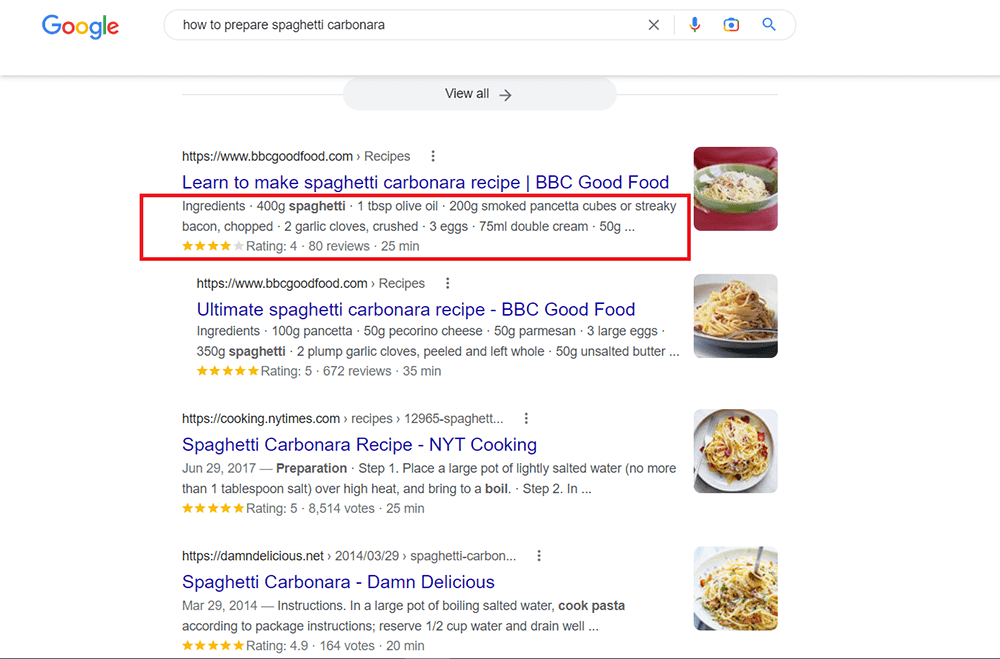The image depicts a Google search results page for the query "how to prepare spaghetti carbonara." At the top of the page, the search bar contains the query text. Just below the search bar, there is a button labeled "View All." 

The primary search result is from www.bbcgoodfood.com, featuring a hyperlink that reads, "Learn to make spaghetti carbonara - BBC Good Food." A small thumbnail image shows a green plate with a spaghetti carbonara dish, placed on a red tablecloth. 

Accompanying the recipe link, a red rectangular box highlights the list of ingredients and some additional information. The listed ingredients are: 400g of spaghetti, 1 tablespoon of olive oil, 200g of smoked pancetta cubes or streaky bacon (chopped), and 2 crushed garlic cloves. The ingredients list continues with 3 eggs, 75 milliliters of double cream, and 50g of an unspecified ingredient.

The recipe has a rating of 4 out of 5 stars based on 50 reviews, and the total preparation time is indicated as 25 minutes.